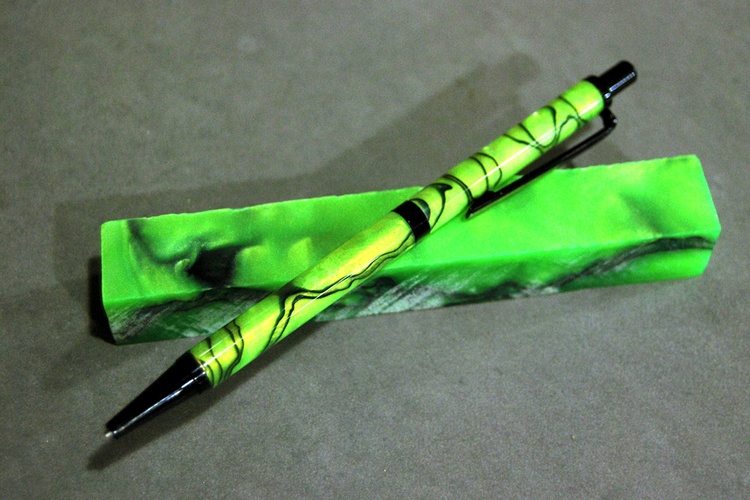The image depicts a bold, neon green ink pen adorned with black marbling and accents. The pen's design features a black click mechanism, a clip, and a black point, and it has a thick black bar in the middle. The glossy, marbled pattern of the pen is mirrored by a matching rectangular block upon which it rests. This block also has a neon green base interspersed with black liquid-like designs. Both objects are centered on a flat surface covered with a short, soft grey carpet, which has visible white specks and dirt scattered throughout. The lighting in the image comes from the right, casting subtle shadows on the left, enhancing the visual contrast between the vibrant pen and its subdued background.